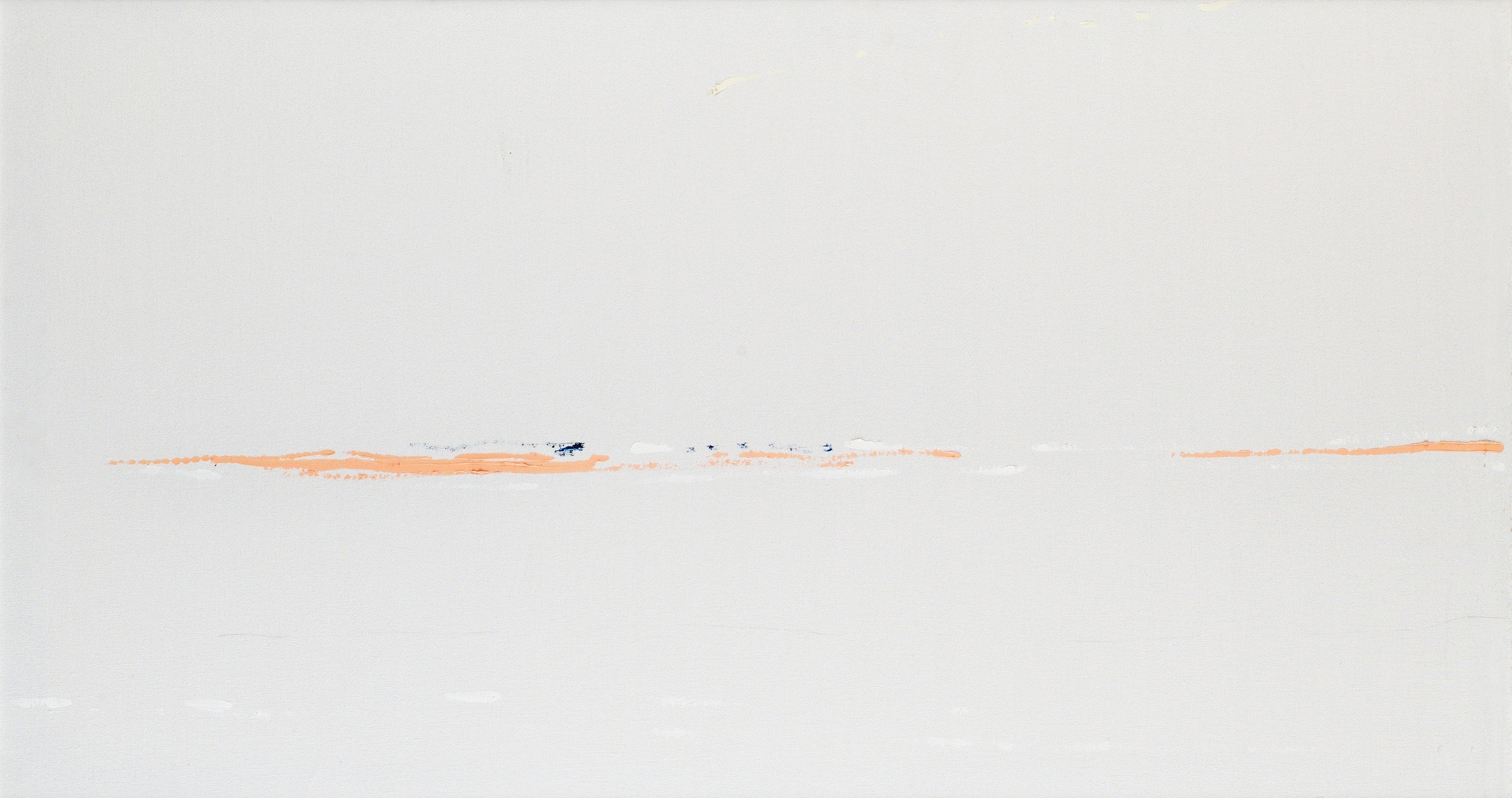The image portrays an abstract, minimalist painting characterized by an expansive, off-white or light gray canvas that dominates the background. The canvas features a single, uneven, salmon-pink line that traverses horizontally across the lower half, slightly below the midline, evoking a sense of interrupted motion with its varying thickness—it begins thin on the left, gradually thickens, and then tapers back to thinness towards the right. This line is accented with subtle, brighter white highlights and small splotches of blue near its beginning portion. Additionally, there are dark splotches interspersed near the line in certain areas, adding hints of complexity to the otherwise stark and empty composition. The overall effect is reminiscent of a serene yet desolate landscape, perhaps suggesting a horizon on a cloudy day with traces of snow and water.